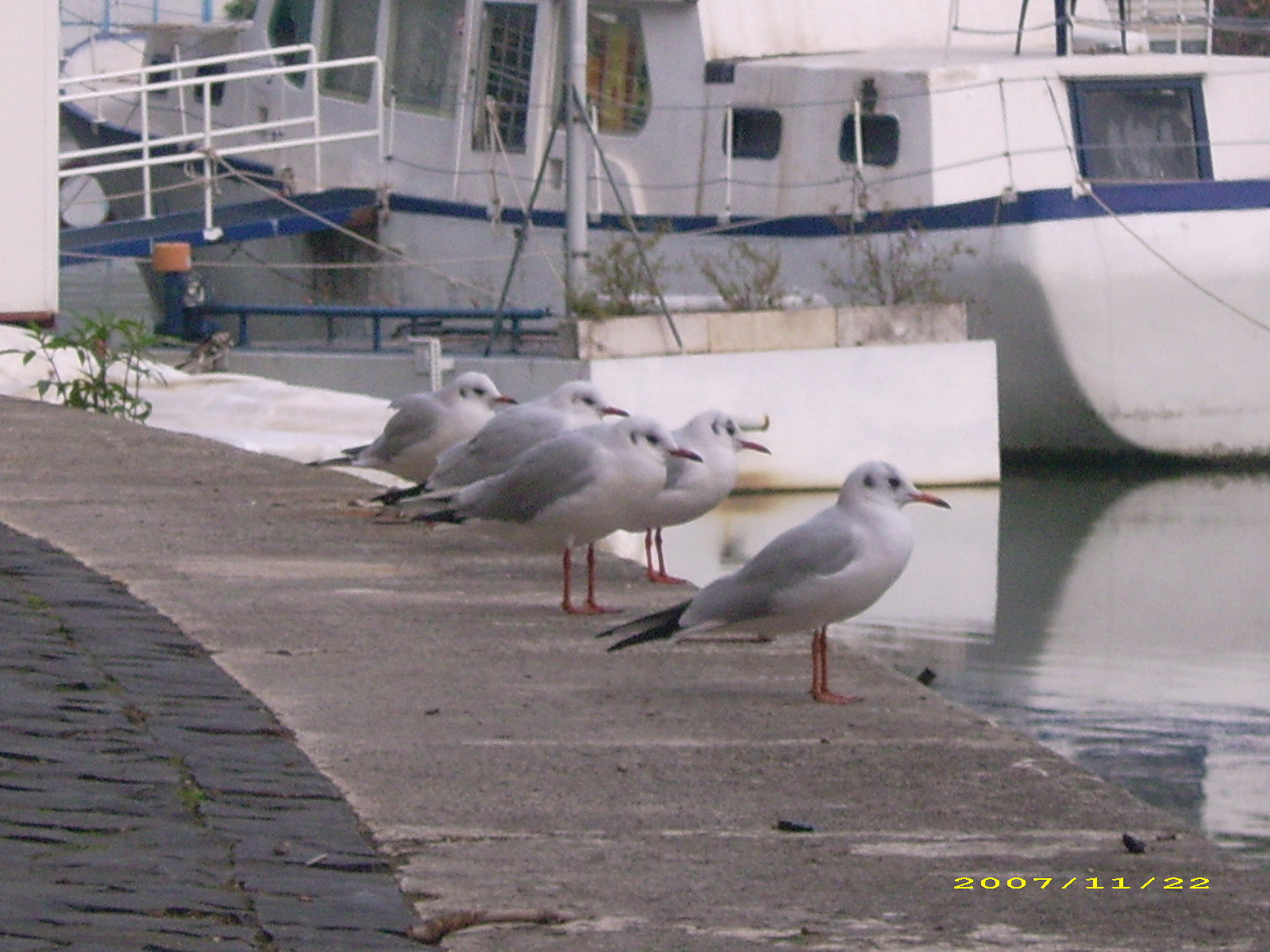The photograph, dated November 22, 2007, depicts a quintet of seagulls standing at the edge of a concrete and cobblestone sidewalk by a body of water, likely a harbor. The seagulls, characterized by their primarily white plumage, gray wings, and black-tipped tails, also feature bright orange beaks and legs. They appear to be squawking and gazing out towards the water, which is to the right side of the image. In the background, a white boat with blue details, including a window with a blue frame and a bridge with blue flooring and white rails, can be seen. The setting suggests a boat yard or marina, with additional boats and bridges visible in the distance.